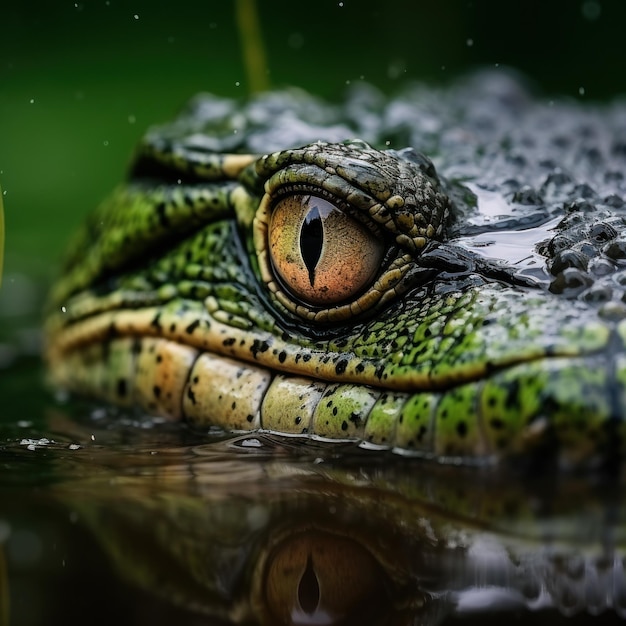The image is a very close-up, full-color photograph of a reptile, partially submerged in water. The background is blurred with shades of green. The reptile, which could be an alligator, crocodile, caiman, or a similar creature, dominates the frame with its head emerging from the water. The visible eye is striking, yellow with a vertical black pupil. The skin of the reptile is predominantly green with black speckles and yellow markings. The green skin transitions to bright green at the nose tip and fades to yellow further back. Black dots are scattered across the green and yellow parts, and the top of the head appears very dark green to black. There are notable water droplets on its head, adding texture to the scales, and its reflection is clearly visible in the water below. The reptile's head is slightly turned, making only the right half visible, while the left half is cut off on the right side of the picture. The water beneath is dark, mirroring the details of the creature's upper face.